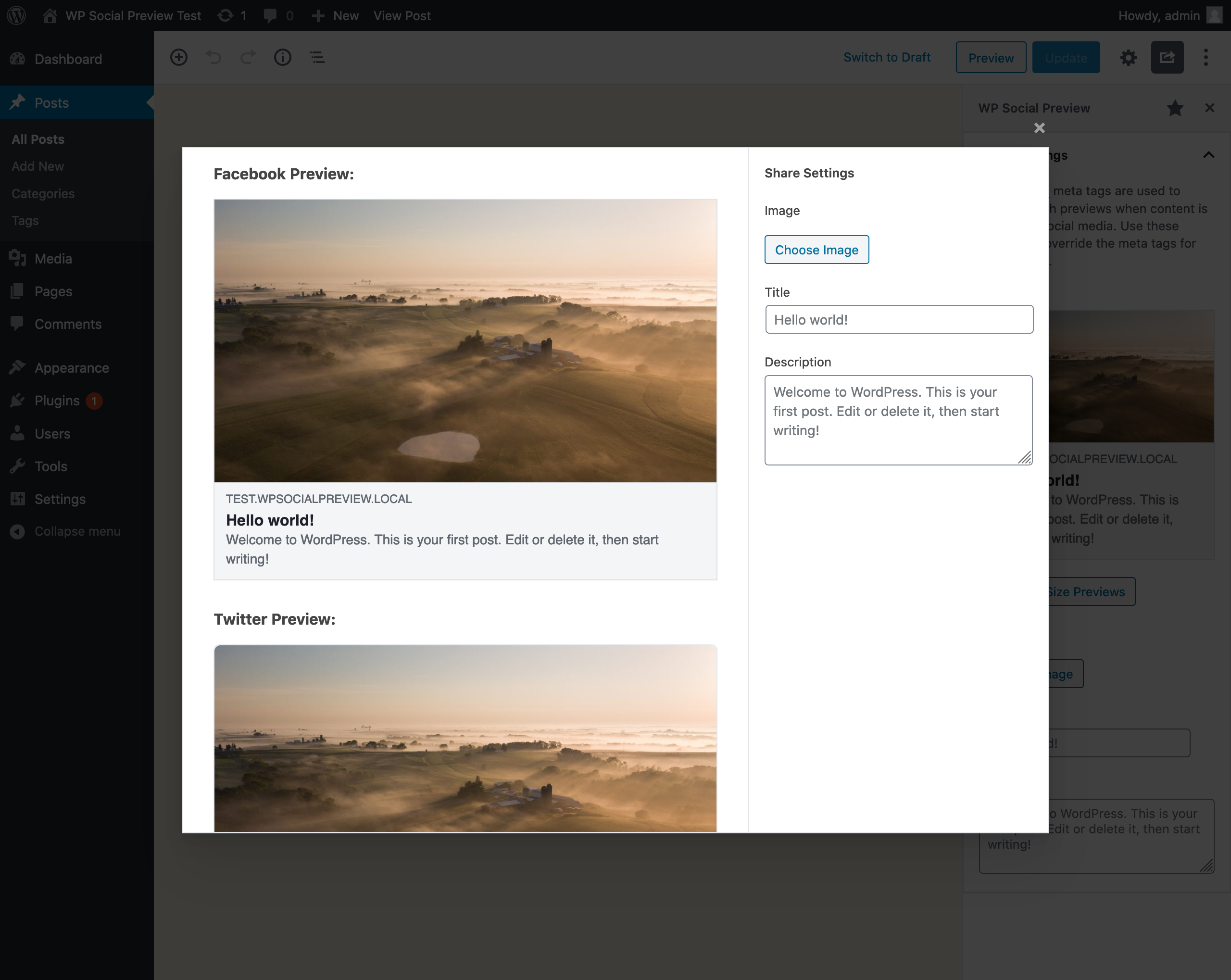The image depicts a web interface with a blurred and grayed-out sidebar on the left. The sidebar contains a column listing options such as Dashboard, Posts, Categories, Tags, Media, Pages, Comments, Appearance, Plugins, Users, Tools, Settings, and a collapsed menu. On the right side, although the text and photos are not clearly visible, there is a prominent pop-up box with a white background labeled "Facebook Preview." This box displays a barren desert scene with text stating "test.wpsocialpreview.local" and "Hello World, welcome to WordPress. This is your first post. Edit or delete it and start writing." Below this, there is a similar "Twitter Preview" showing the same desert image. The interface also includes a section labeled "Share Settings," featuring a blue "Choose Image" button, and text fields for "Title" and "Description." The title field contains "Hello World," and the description field reads "Welcome to WordPress. This is your first post. Edit or delete it and start writing."